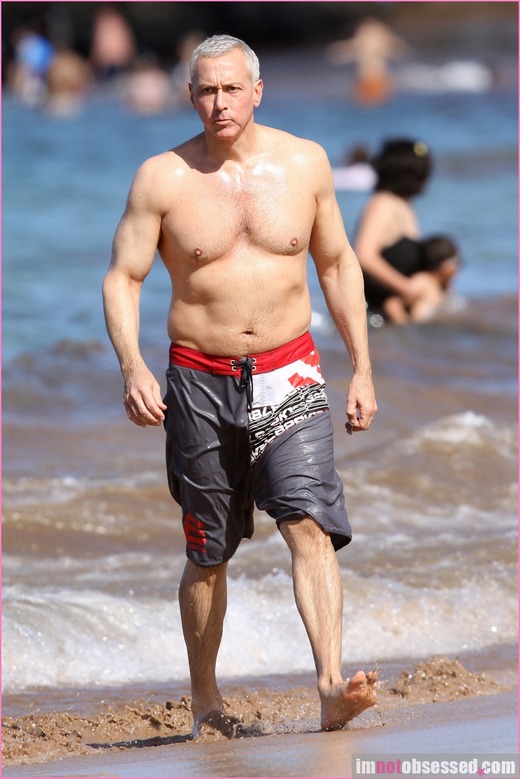This image captures a man with gray hair, resembling Mike Pence, walking on a sandy beach area as he emerges from the water. He is wearing swim trunks featuring a pattern of gray, white, and red, with no shirt, shoes, or socks. The swim trunks are visibly wet, emphasizing that he has just come out of the water. The man appears to be muscular and in good shape, with defined musculature and no noticeable fat. His hair is parted to the side, and he is clean-shaven. In the out-of-focus background, several people can be seen in the water, including someone giving a piggyback ride. The scene suggests it's a lake, as there are indistinct signs of vegetation or a building in the distance rather than an open ocean view. At the bottom right of the image, there is a watermark reading "I am not obsessed dot com" in mostly white letters, with the "O-N-O-T" and the period before "com" in pink.